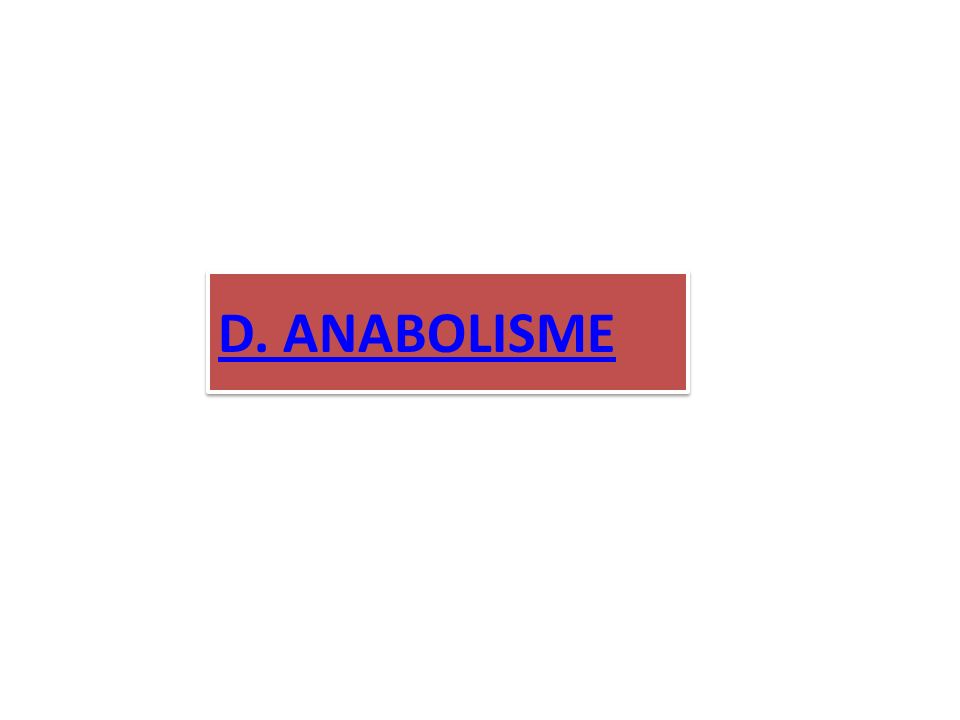The image displays a nameplate, possibly affixed to a door, with a brick-red background. The name "D. Anabolisme" is prominently featured in large, uppercase letters utilizing a blue font. The name reads "D. Anabolisme" with a period after the "D," and "Anabolisme" is spelled A-N-A-B-O-L-I-S-M-E. This name is underlined with a dark blue, bold line, adding emphasis. The nameplate itself is a small, horizontal rectangle.